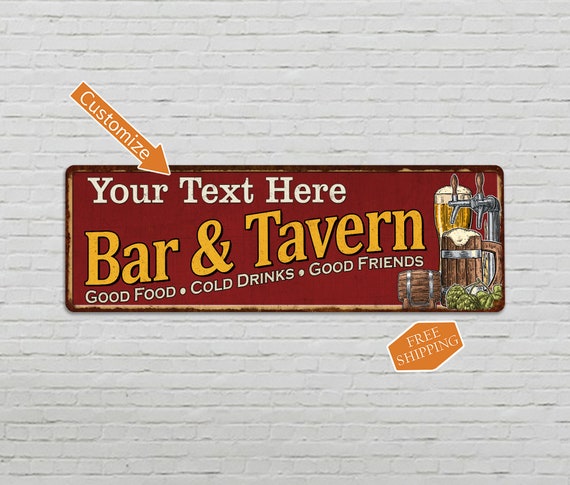The image showcases a detailed mock-up of a customizable bar sign mounted on a white-painted brick wall. The sign, designed to evoke a vintage aesthetic with its rusty border, is a horizontally oriented metal rectangle with rounded corners and a deep red background. Dominating the top left in large white text is a customizable space labeled "Your Text Here," followed by a wave-patterned, prominent yellow text outlined in black that reads "Bar and Tavern." Below this, smaller white text continues in the same wave pattern, stating "Good Food, Cold Drinks, Good Friends." The right side of the sign features detailed illustrations, including a bar tap, a frosty pint glass, a wooden beer mug, and a small beer cask. Above the sign, an orange arrow with a white outline and white text proclaims "Customize," while the bottom showcases an orange hexagonal badge with a white outline that reads "Free Shipping." The overall design resembles a vintage, elongated license plate, and the depicted items such as hops, barrels, and beer taps emphasize its theme.